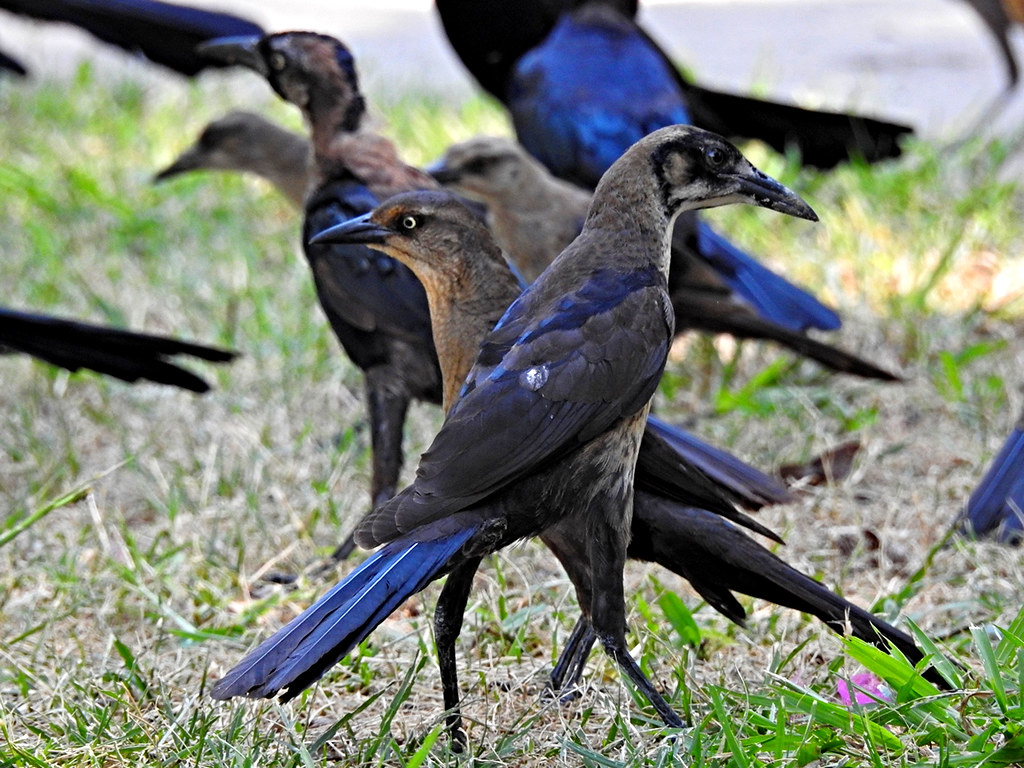This image captures a group of birds standing on a patch of grass that is a mix of green and brown, suggesting it's somewhat dried out. Central to the image are five birds arranged in alternating directions, with the closest bird facing right and the others primarily facing left. These intriguing birds boast distinct features: their bodies are mostly brown with some areas of black, their beaks, eyes, and legs are black, and they are adorned with vibrant blue tail feathers and patches of blue and gray on their wings. One bird in the foreground presents a clear side profile and even has a small bird dropping on its wing. In the background, the scene is bordered by a cement-colored sidewalk, indicating a park setting. Additionally, there is a pink object—possibly a flower or piece of trash—visible in the bottom right corner of the image. The birds appear calm, comfortably standing and interacting within their grassy habitat.